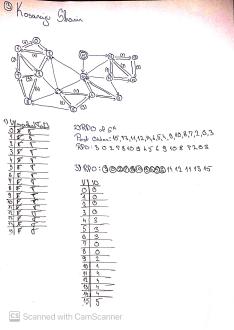A small digital scan of a photograph of a piece of paper, marked at the bottom with "scanned with CAM scanner." The paper has a distinct pinkish hue along the top edge, with the remainder being predominantly white. In the top left corner, there is a small happy face drawn, and below it, a handwritten name in script, possibly reading "KOSAIGO SHAIN." Below the name, a detailed chemical structure is depicted, consisting of connected lines and circles, each circle containing numbers. Further down, there are several tables; the first table on the left starts with the number zero and continues sequentially up to fifteen. To the right side of the page, some columns appear to show the letters "F" and "T," potentially indicating "False" and "True," although the exact context is unclear.